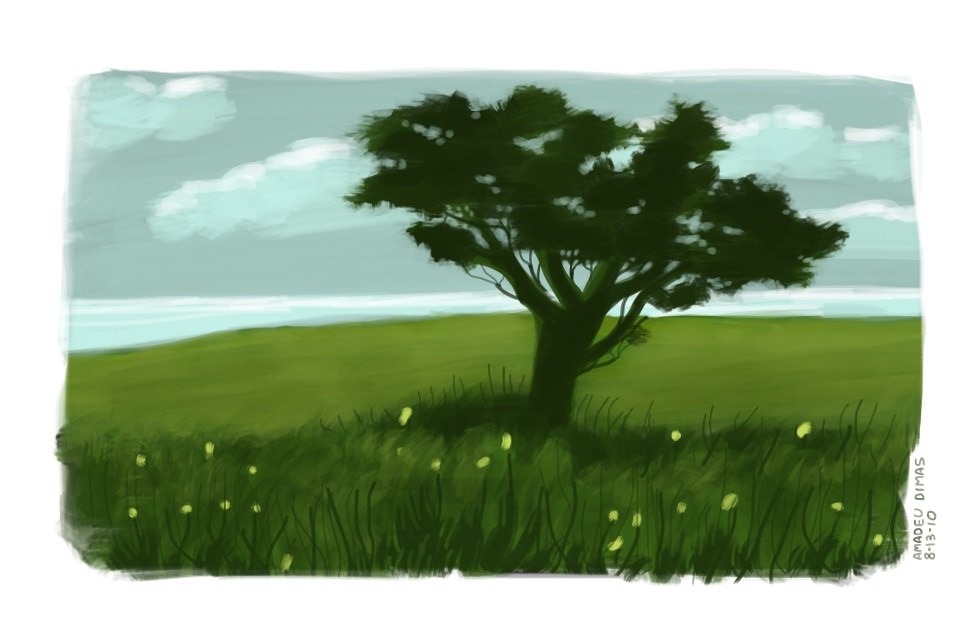This horizontally oriented color painting depicts a tranquil landscape featuring a single, distinctive tree in the middle of an expansive green field. The composition is rich with various shades of green, from the bright greens of the vast field to the darker greens of the foreground grass. The grass at the bottom of the image is dotted with yellowish-white spots that could represent flowers or possibly fireflies, enhancing the serene atmosphere. The tree, centered in the field, has a dark trunk with leaves that branch out and resemble broccoli in their shape and texture. The sky above is a flowing grayish-blue with fluffy clouds highlighted in white at the top, presenting a peaceful backdrop. Just above the horizon line, where the field meets the sky, there is a hint of a body of water, adding depth to the scene. The bottom right-hand corner of the painting contains the artist's name, "Mando Dimas," followed by the date "8-13-10," written vertically. The overall effect is a serene and picturesque landscape that captures a moment of natural beauty in a slightly hilly, yet predominantly flat, green terrain.